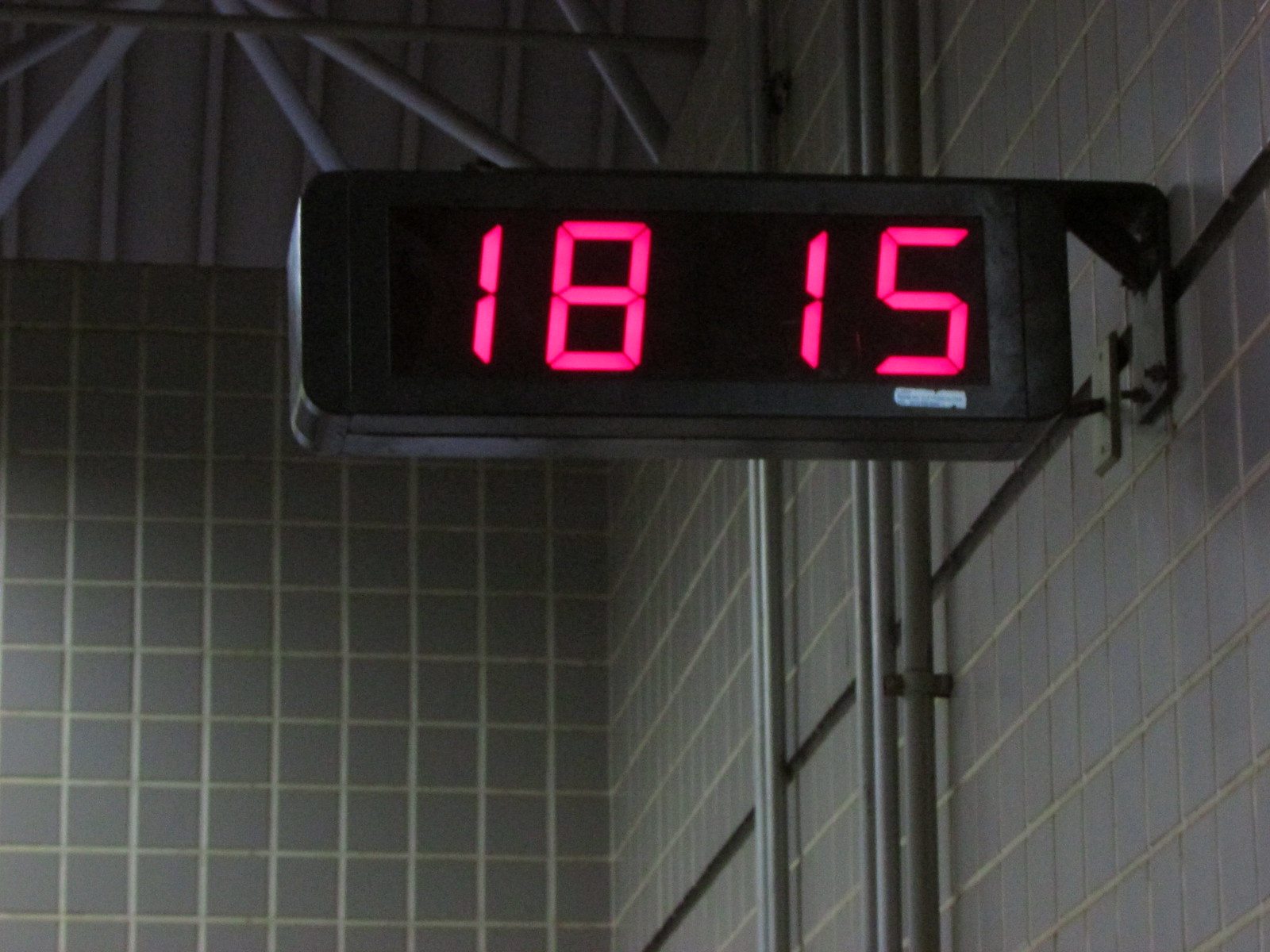The image depicts a large black digital sign mounted perpendicularly to a towering gray tiled wall with light gray grout. The wall, likely part of a spacious public space such as a bus terminal or train station, features various vertically oriented gray pipes. The ceiling soars high above, adorned with dark gray cylindrical beams. Central to the image, the digital sign displays the numbers "18 15" in bright red, blocky digits reminiscent of those on old digital clocks. The sign also bears some additional white writing below the digits, which appears unclear in purpose. Off to the bottom left, subtle illumination hints at possible daylight filtering in from outside. The overall composition is in landscape format and captured in color, providing a comprehensive view of this public indoor setting.